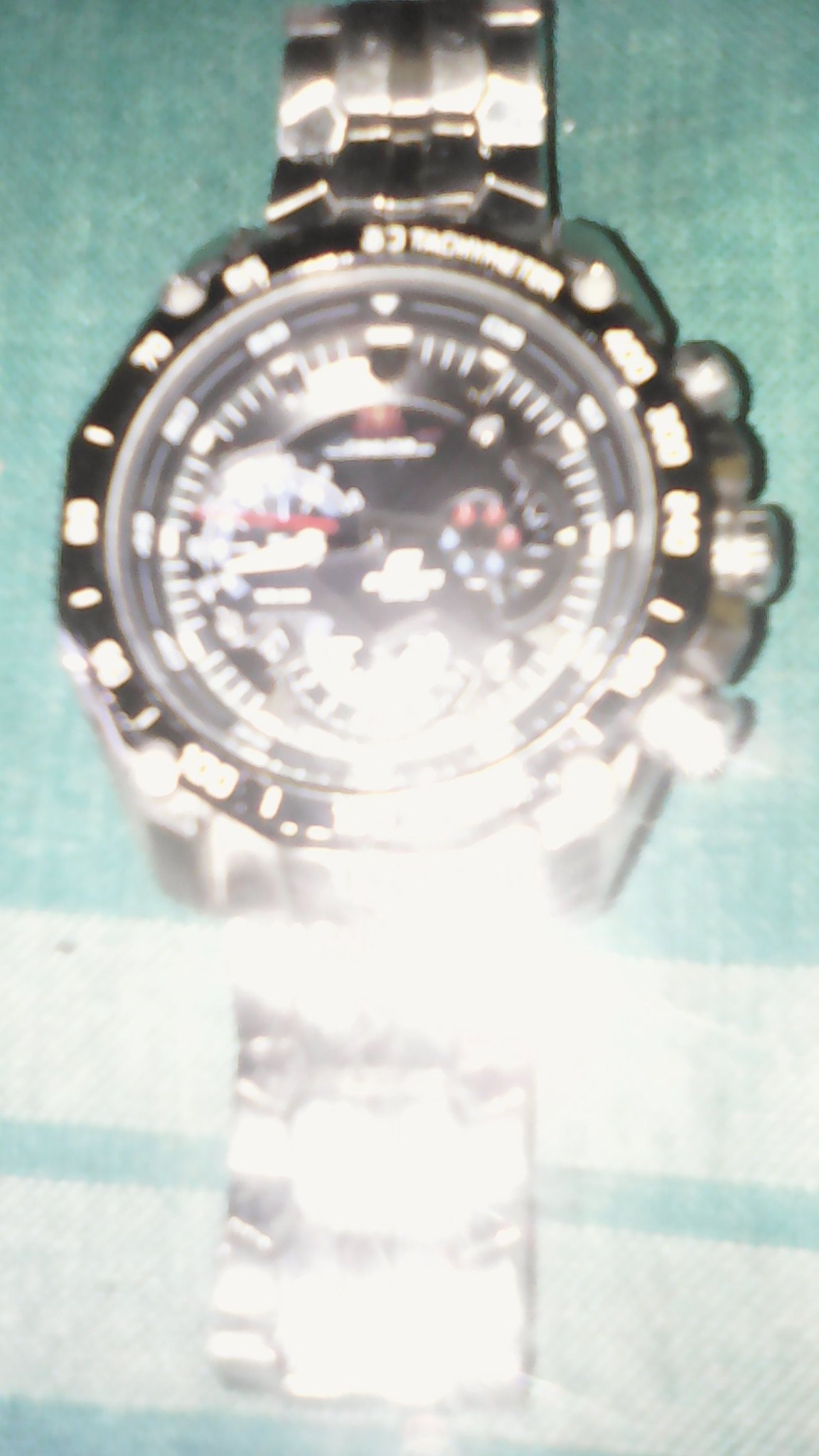This photograph captures a silver wristwatch positioned on a green background that gradates to a lighter green, with two wide horizontal white stripes at the bottom quarter. The watch, which features a stainless steel wristband, is illuminated by a strong light that creates a significant glare, obscuring many details. The watch's round face, made of glass, showcases a black bezel and black inner face with white time markings. Additional features include a red hand pointing towards the 9 o'clock position, and a complex central area with smaller dials and dots—three red and three blue on the right side. The center also appears to have a red element with a yellow inner section at the top. On the outer edges, the watch displays a winding shaft with two small adjacent buttons on the right side. The intense glare from the light source blurs the lower half of the image, making specific details challenging to discern.